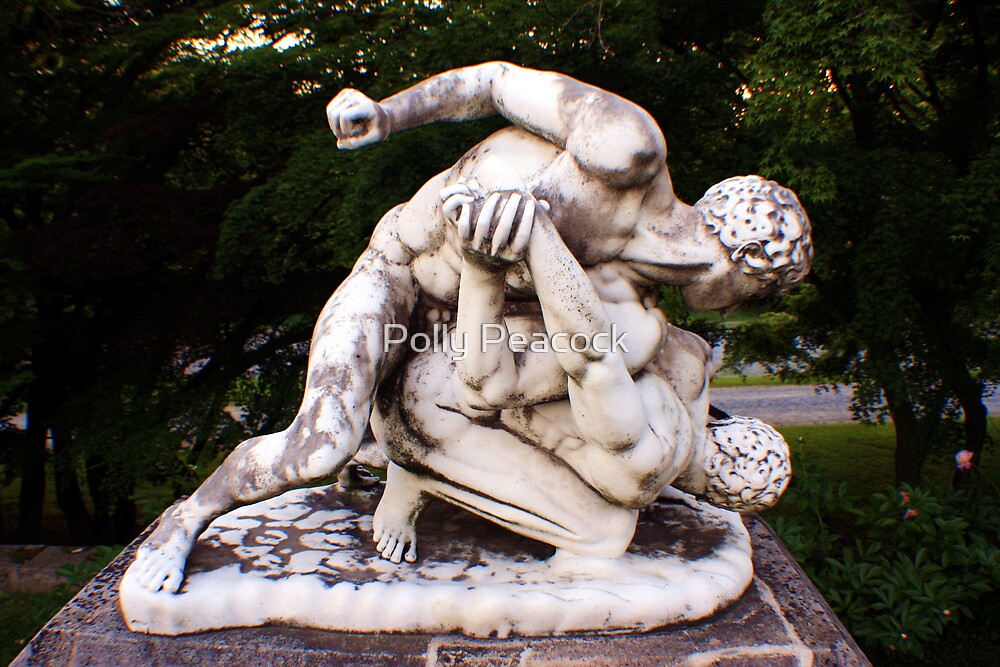In the photograph, there is a Greco-Roman style marble statue depicting two muscular, naked men wrestling. The dominant figure, positioned on top, has his right hand extended back in a punching motion, while his feet pivot in that direction, suggesting imminent physical action. The man beneath, crouched and shielding himself, seems to be at a disadvantage, with his head towards the base of the statue. The statue has weathered over time, evident from the dirty gray splotches marring its surface. It stands on a rough, rectangular stone base. Surrounding the statue is a verdant outdoor setting; to the right, a large-trunked tree extends its branches overhead, casting a network of shadows, while to the left, another substantial tree mirrors this arboreal frame. Beyond the immediate grassy patch with trees, a road is visible in the distant background, indicating the statue’s placement in a park-like environment.